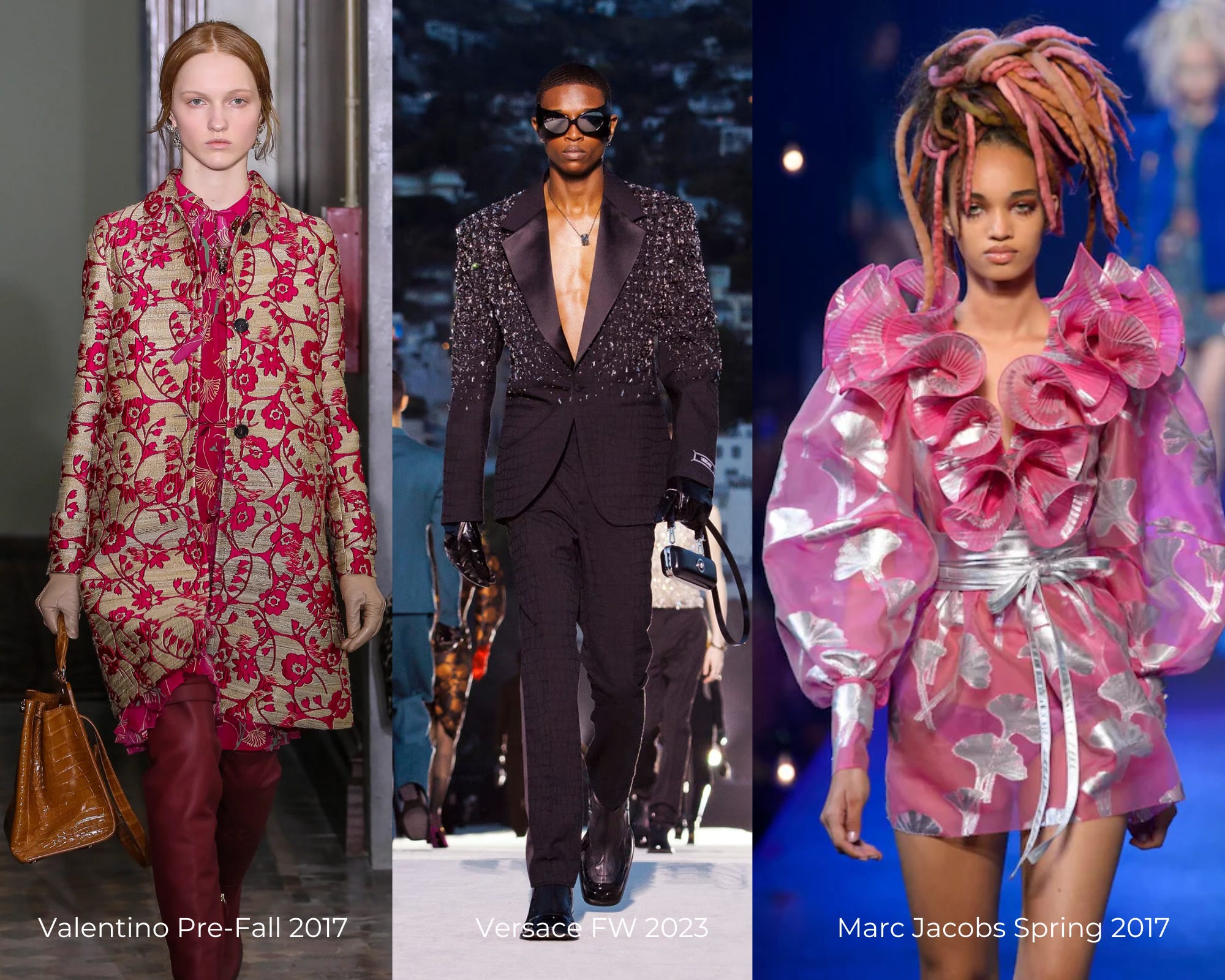The image showcases three striking models side by side, each representing different high-fashion designers. At the bottom, the text highlights "Valentino's Pre-Fall 2017," "Versace FW 2023," and "Marc Jacobs Spring 2017."

On the left, a young Caucasian woman, approximately in her mid-20s, sports brownish-red hair. She is clad in a chic blend of a pink dress and a gold jacket, intricately designed with both pink and gold patterns. Accessorizing her outfit, she carries a brown bag and wears tall maroon boots or possibly tights. Her expression is serious as she poses on the runway.

In the middle stands an African-American man with short black hair, wearing an exquisite black suit adorned with sparkling details at the top. The suit is worn without a shirt underneath, exposing his chest and adding a bold edge to the ensemble. He complements his look with black sunglasses, exuding confidence and style.

On the right, a young African-American woman with a radiant light brown complexion features her multicolored dreadlocks—an artistic mix of dark brown, pink, light brown, lavender, yellow, and silver. Her dress is a vibrant pink with silver floral designs, featuring a ruffled neckline and voluminous sleeves that taper at the wrists. She cinches the outfit with a silver ribbon belt at the waist, adding a touch of elegance to her striking appearance.

All three models convey high fashion through their distinctive and diverse styles, epitomizing the essence of the renowned designers they represent.